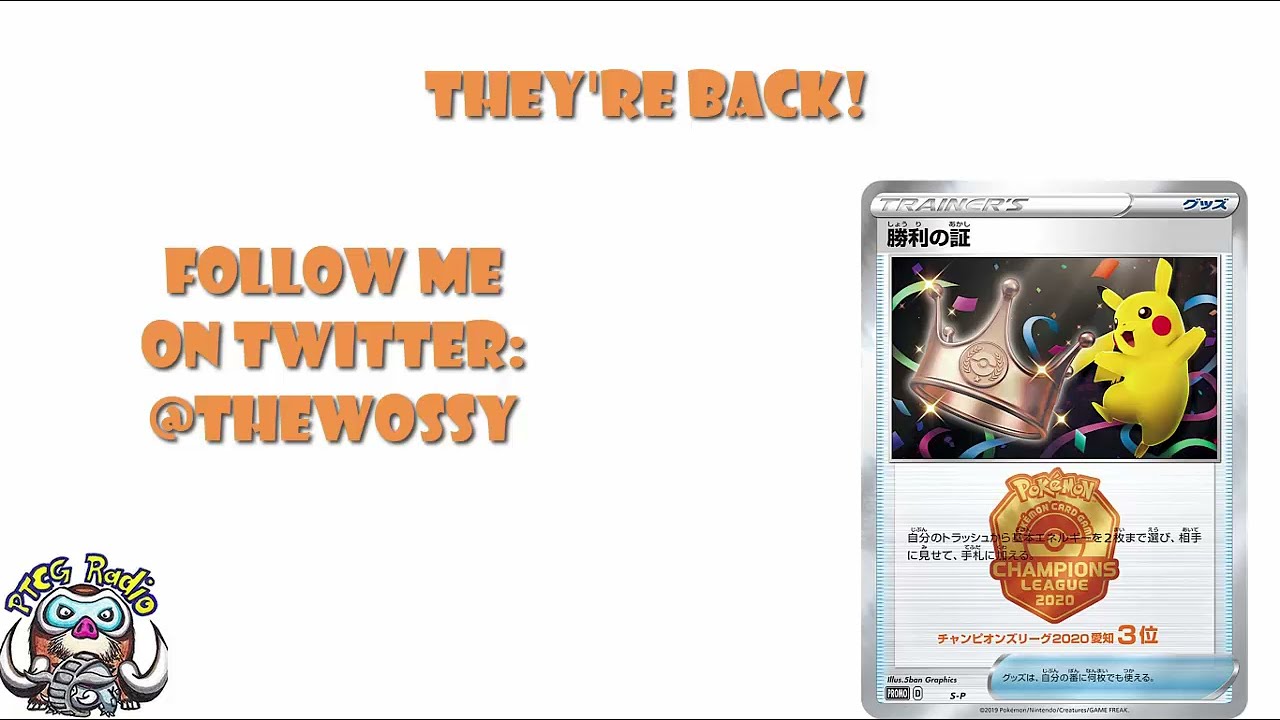The image prominently features a Pokemon card set against a white background with various elements overlaid. The top of the image reads, "They're Back!" in vibrant orange text, followed by a call-to-action, "Follow me on Twitter: @TheWossi", in the lower left region. The Twitter handle is spelled "T-H-E-W-O-S-S-Y". The bottom left corner of the image showcases a playful logo for "PTCG Radio", featuring a cute mascot that appears to be wearing a mask and goggles, potentially a stylized creature resembling a cartoonish beaver or chipmunk.

The centerpiece of the image is a Japanese Pokemon card for the Pokemon Champions League 2020, featuring Pikachu prominently. Pikachu, the iconic yellow Pokemon with big black-tipped ears and red cheeks, is depicted dancing with a gold crown to its left. The card is set against a festive black background with colorful confetti, all beneath the overarching banner headline in orange. The entire composition appears to be a well-crafted advertisement, possibly created on a computer, designed to engage viewers with its inviting and playful design.